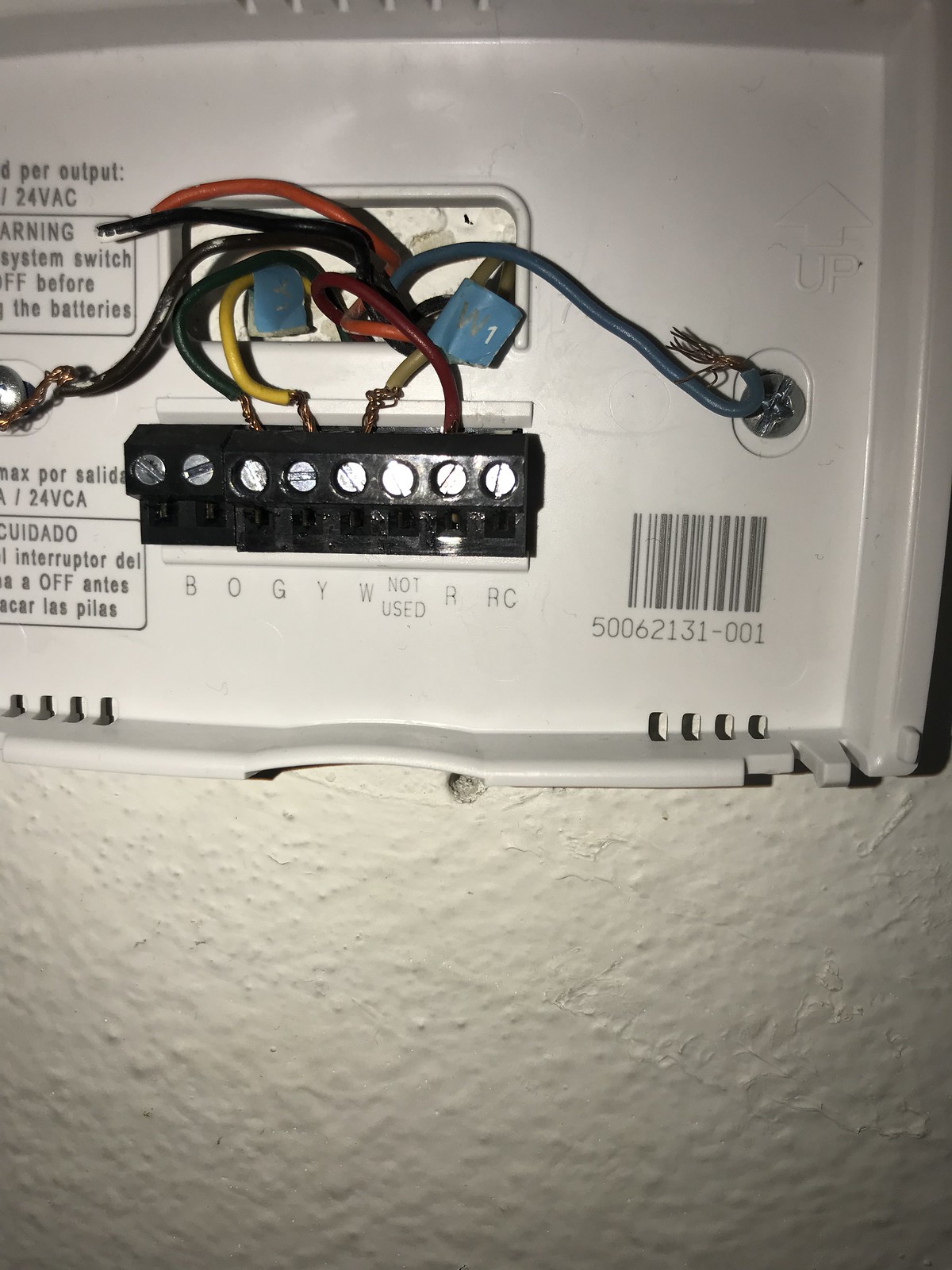The photograph depicts a white wall mounted with an intricate electronic device. This device is prominently connected to a network of various colored wires, including black, green, yellow, orange, red, and blue. Two of the yellow wires are marked with blue tape labeled "W1." The wires are affixed to a black connector secured by eight silver screws. The screws are labeled from left to right as follows: B0/O, G, Y, W, not used, R, and RC.

Adjacent to the connector, a barcode is visible with the number "50062131-001" underneath it. Above the barcode, an arrow pointing upwards is accompanied by the word "UP." The left side of the device features several inscriptions, among them: "D per output; 24VAC," and inside a square label, "WARNING: System switch OFF before the batteries."

Further inscriptions to the left of the black connector read, "NAXPORSOLIDA/24VCA," and within another square, "SUADADO, INTRUDERDEL, A OFF ANTES ACAR LAS PILAS." The entire device is set against a white background, giving it a clean and technical appearance.